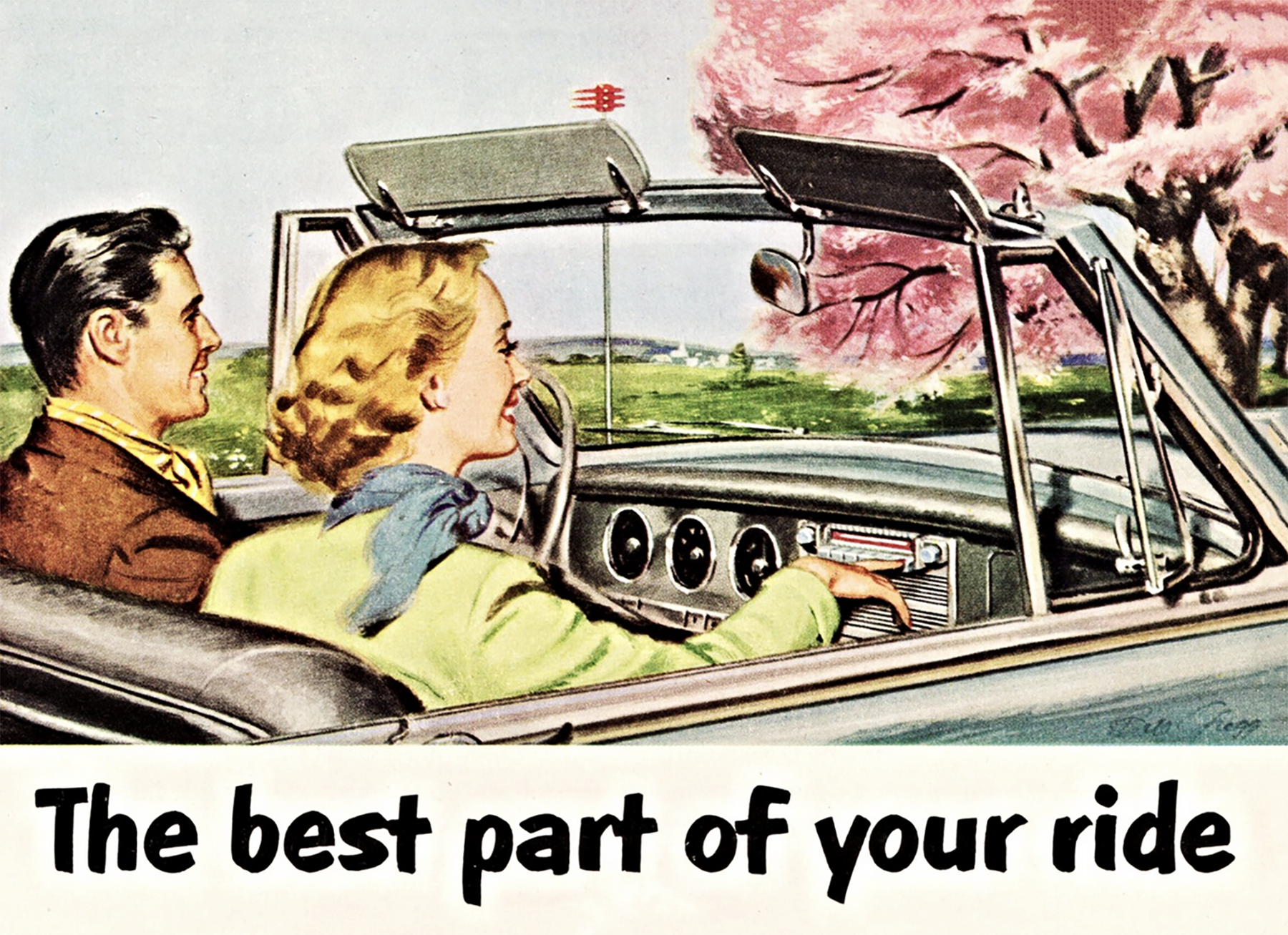The image is a vintage 1950s-style artwork depicting a cheerful couple in a convertible car, reminiscent of classic advertisements from that era. The scene shows a man in the driver's seat on the left, captured in profile with slicked-back dark hair, wearing a brown suit and a yellow cravat. Beside him, on the right, sits a woman with short, lightly waved blonde hair, dressed in a lime green dress or jacket paired with a blue scarf around her neck and wearing lipstick. She is reaching over to the car radio, pushing one of the buttons. Both individuals are smiling as they drive along a scenic route with green hills, a blue sky, and a distinctive tree with pink leaves visible in the background. The artwork, rendered in a detailed, colored pencil style, is captioned at the bottom in black lettering: "The Best Part of Your Ride."